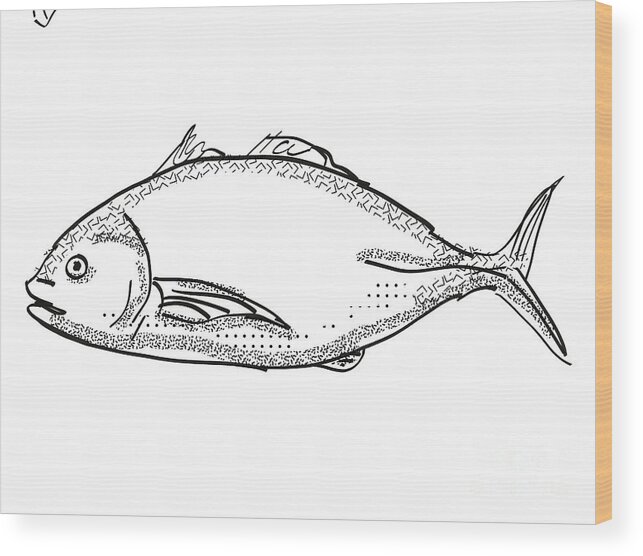The image depicts a rectangular canvas with a wooden frame, where the darker gray canvas front exhibits a meticulously crafted sketch of a fish rendered in black ink or pen. The fish, outlined in rich black with some shading work, primarily occupies the middle two-thirds of the canvas, presenting a side view with its head on the left and its tail on the right. The body of the fish features detailed elements, including one pronounced eye, a relatively short back fin, very small side fins, and an L-shaped pattern near the top portion of its body. The fish's fins are distributed with two at the top and one at the bottom, while additional small and large dots adorn the fish's body, adding to the intricacy of the sketch. The edge of the wooden frame is light brown, contrasting with the whitewashed finish of the wood behind the drawing, allowing the darker gray color of the canvas and the black sketch to stand out prominently. This artwork, likely a canvas print, does not include any text, ensuring that the focus remains solely on the striking fish illustration.